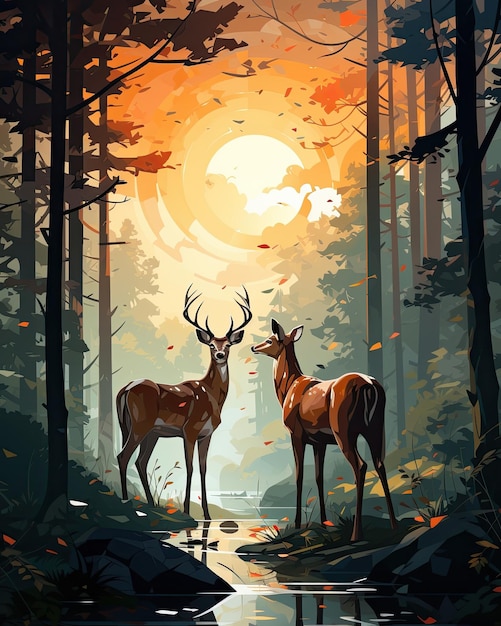The painting depicts a serene autumn forest scene, featuring a delicate stream running through its center, bordered by gentle banks. On either side of the stream stand a majestic stag with grand antlers on the left, and a graceful doe on the right. The stag gazes back directly at the viewer, while the doe’s attention is turned towards the stag. Towering, robust trees frame the scene, their leaves cascading down like confetti in rich autumn hues, enhancing the seasonal atmosphere. In the background, a colossal sun dominates the sky, surrounded by concentric rings of vibrant colors ranging from yellows to deep reds and oranges, creating an ethereal glow. The forest stretches out behind the deer, offering glimpses of additional trees mingling into the colorful horizon, evoking a sense of depth and tranquility. It's a beautiful, detailed painting that captures a moment of stillness and natural beauty.